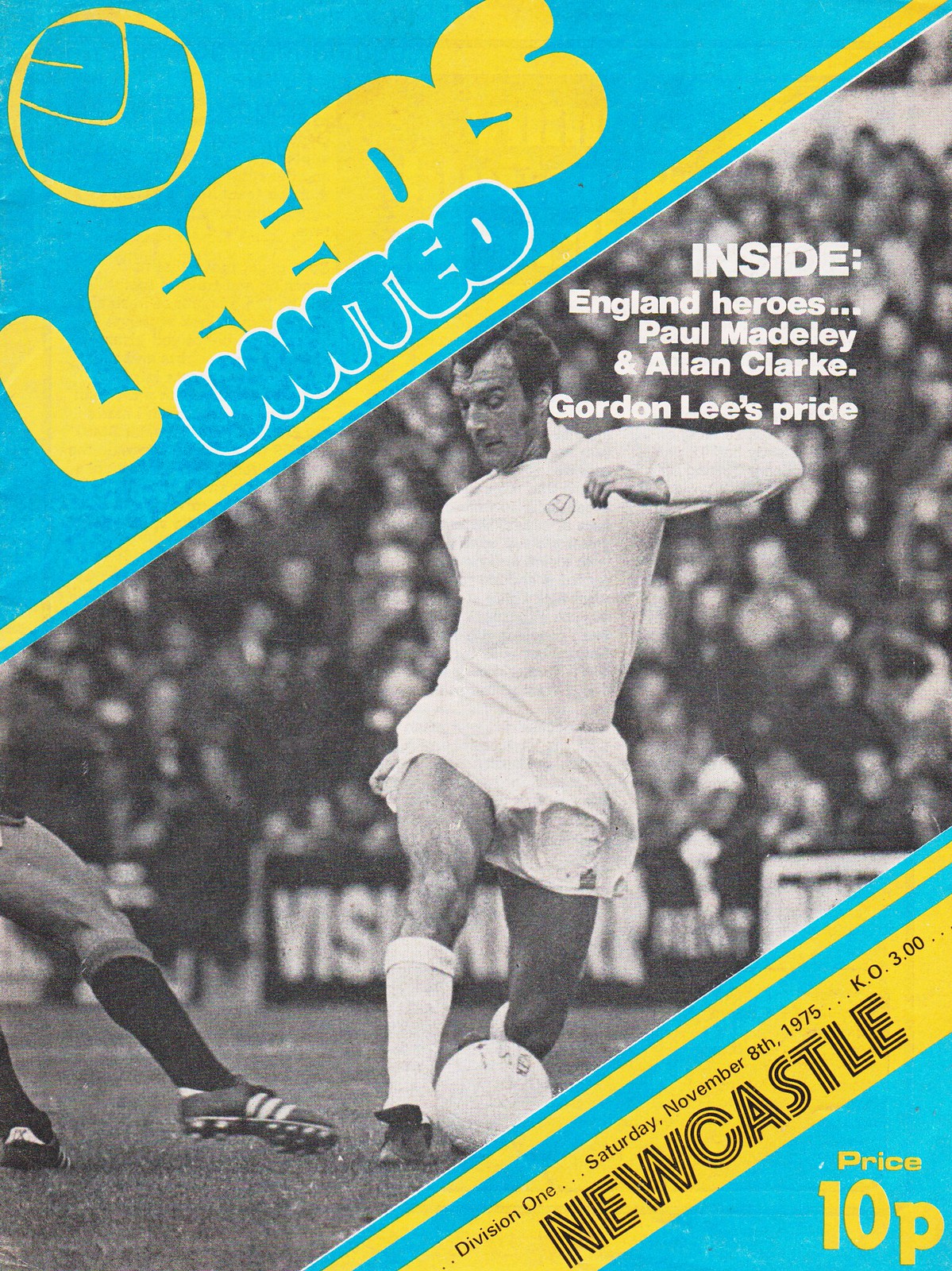The cover of this old magazine, published by Leeds United, prominently features a nostalgic black and white action photograph of a European football player from the 1970s, dribbling a soccer ball while a defender dives in the wrong direction. Dominating the top left corner is the Leeds United title written diagonally in yellow text against a powder blue background with a team logo above it. Centrally positioned atop the photograph is white text that reads "Inside: England Heroes, Paul Madley and Alan Clark, Gordon Lee's Pride." In the bottom right corner, another powder blue background hosts a yellow banner with black text detailing the match information: "Division 1, Saturday, November 8th, 1975, KO 3.00, Newcastle, Price 10p."